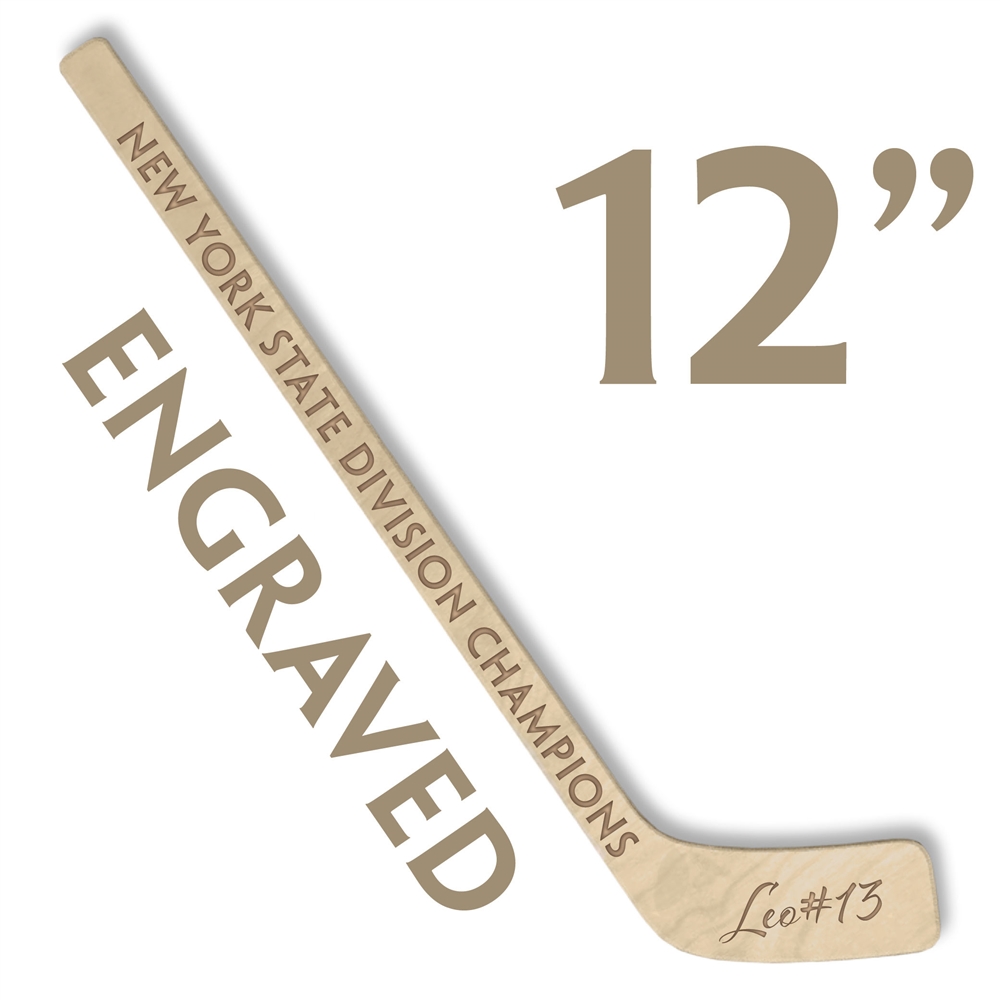The photograph features a simple, light tan hockey stick made from a single piece of wood, set against a white background. The wood exhibits a subtle, almost imperceptible grain, giving it a smooth, lacquered texture. Along the length of the handle, dark brown text is engraved, reading "New York State Division Champions." Near the bottom, where the blade of the stick contacts the puck, cursive engraving displays "Leo No. 13." In the lower left corner, parallel to the stick, bold text in a brown color states "ENGRAVED." Finally, in the upper right corner, large light red text prominently indicates "12 inches."